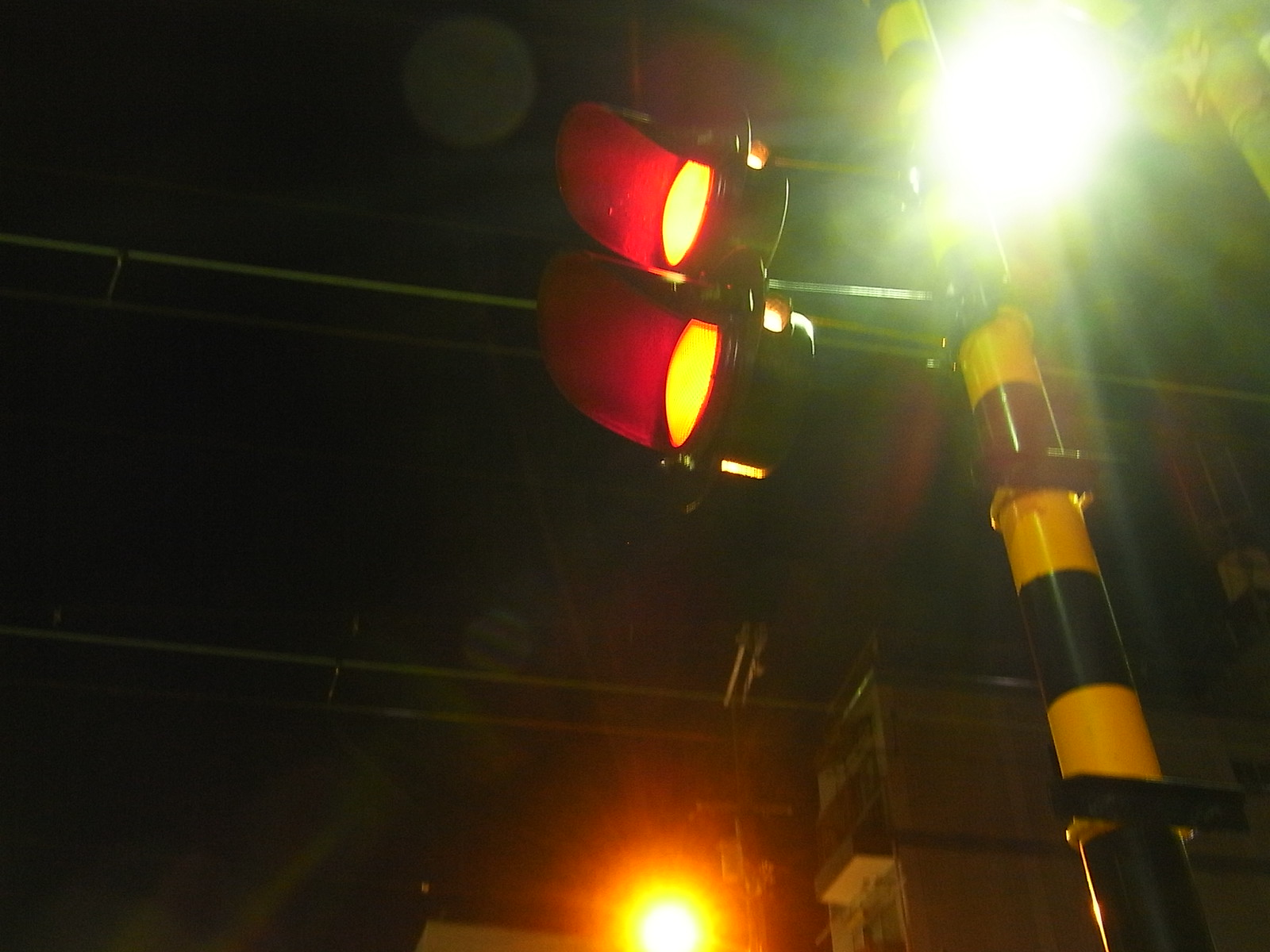A street scene at night captured in this photograph reveals a starkly contrasting environment against a pitch-black sky. Dominating the right side of the image is a large, cylindrical pole crafted from metal. The pole is meticulously painted in alternating stripes of black and yellow, creating a visually intriguing pattern. Ascending the pole, near the top-middle section of the photograph, are two circular orange street lights. These lights are encased in black cylindrical bases, which securely hold the glowing domes within them. Above each light, a black dome encapsulates the illumination, with light reflecting off the dome and casting a reddish hue. In the top-right corner of the image, a dazzling white light shines down brightly, adding an intense glow to the overall composition and altering the perception from which the photograph is taken.